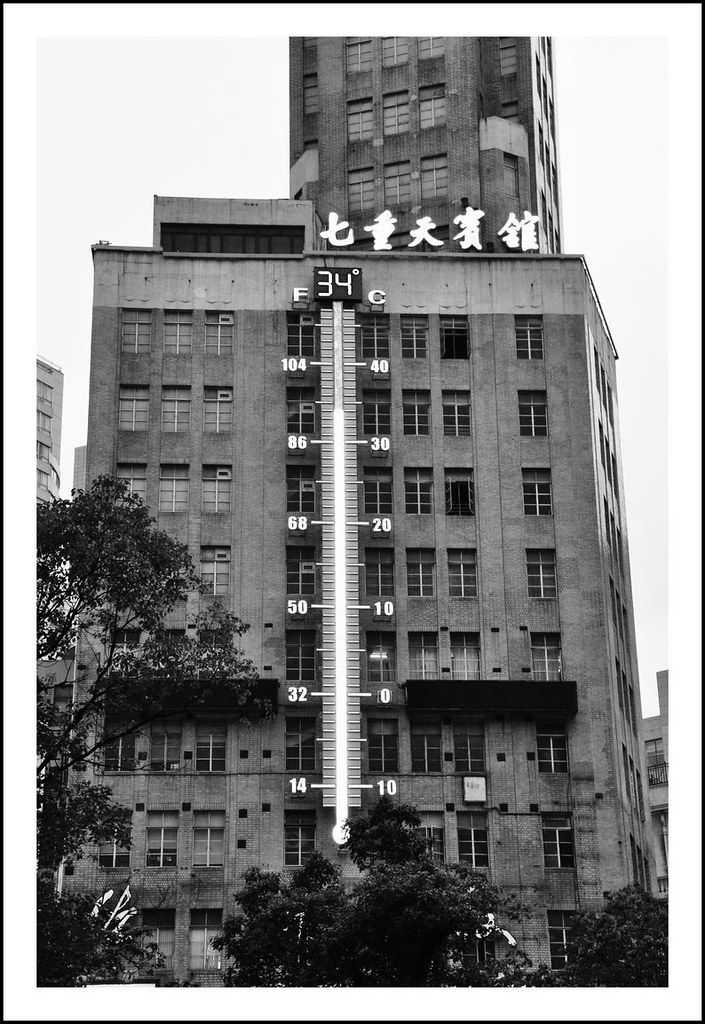This black-and-white photograph captures a tall, intricately detailed brick building in China, as indicated by the prominent Chinese characters displayed in white on the facade. The image is elegantly framed with a thin black border, further accentuated by a white matting. The building itself features distinct concrete trim at the top of each section, adding a refined architectural touch. Above the main structure, a slender tower-like extension rises, also constructed from brick and adorned with numerous windows.

On the top left corner of the building, adjacent to the Chinese characters, there is an additional structure on the rooftop, which appears to house a stairway or serves as an access point. At the base of the photograph, the presence of trees—situated at the bottom left, center, and right—adds a natural element to the urban scene.

A noticeable feature of the building is a fire escape or balcony on the right side. In the center of the main building facade, there is a tall metal thermometer. This thermometer shows a temperature reading of 34 degrees Fahrenheit (noted with an 'F' on the left side) and has a corresponding Celsius scale on the right. The thermometer is a bright silver color with white numerals along its sides, making it a prominent focal point within the composition.